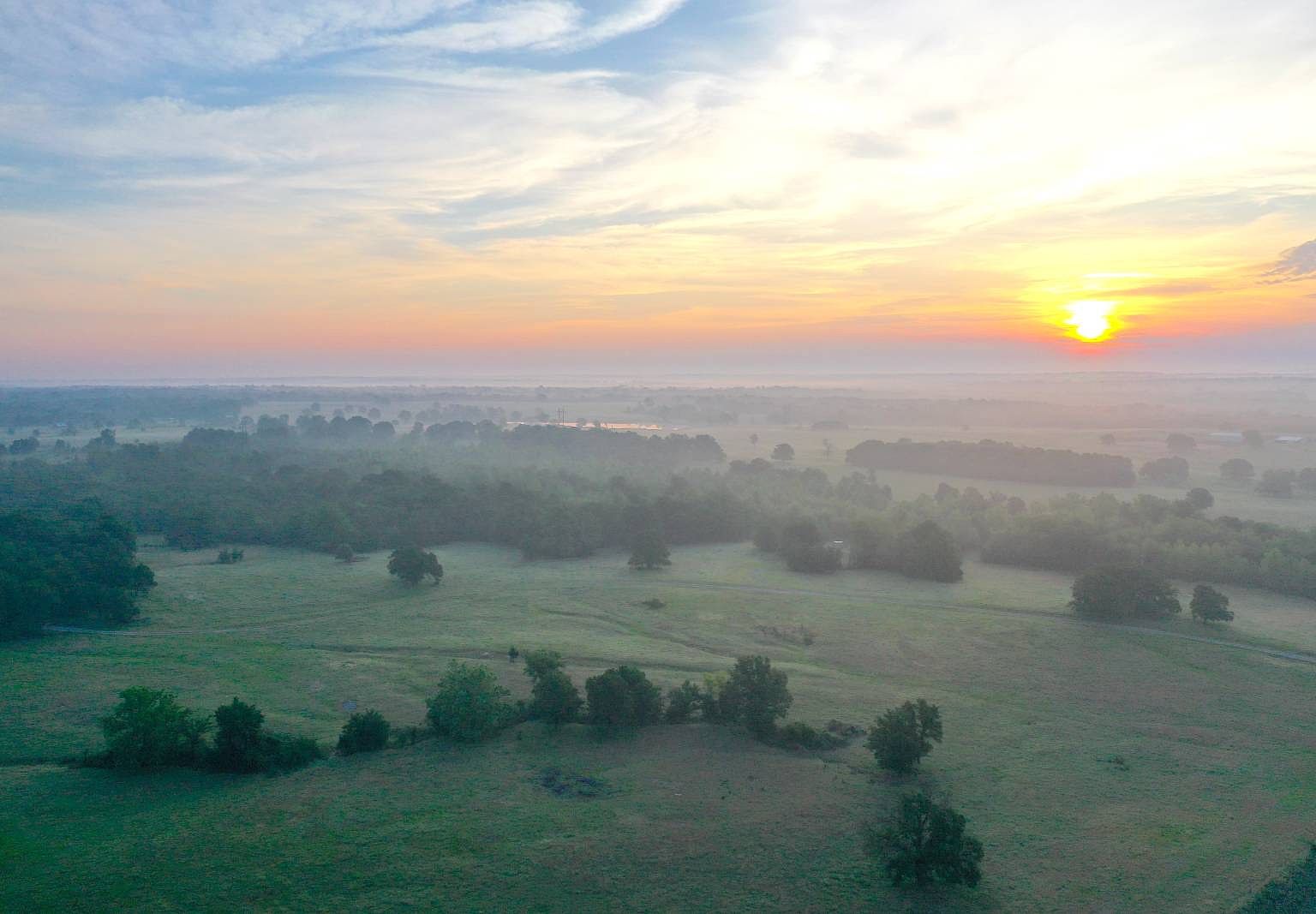The photograph captures a breathtaking aerial view of a vast, pristine natural landscape at sunrise. On the upper right side of the image, the bright white sun is enveloped in a radiant orange glow as it rises from the horizon, transitioning through hues of yellow and orange, casting warm light across the scene. The sky toward the top left of the image is a clear blue, dotted with white clouds. Below, there are streaks of yellow and orange-tinged clouds closer to the horizon. In the middle of the photograph, there is an extensive grassland densely populated with tall, green trees. Near the bottom of the image, a row of shorter trees lines the foreground. Scattered throughout the green fields are small bushes and natural paths, emphasizing the untouched beauty of the landscape. A light fog hangs over the ground, giving the scene a serene, almost mystical atmosphere.